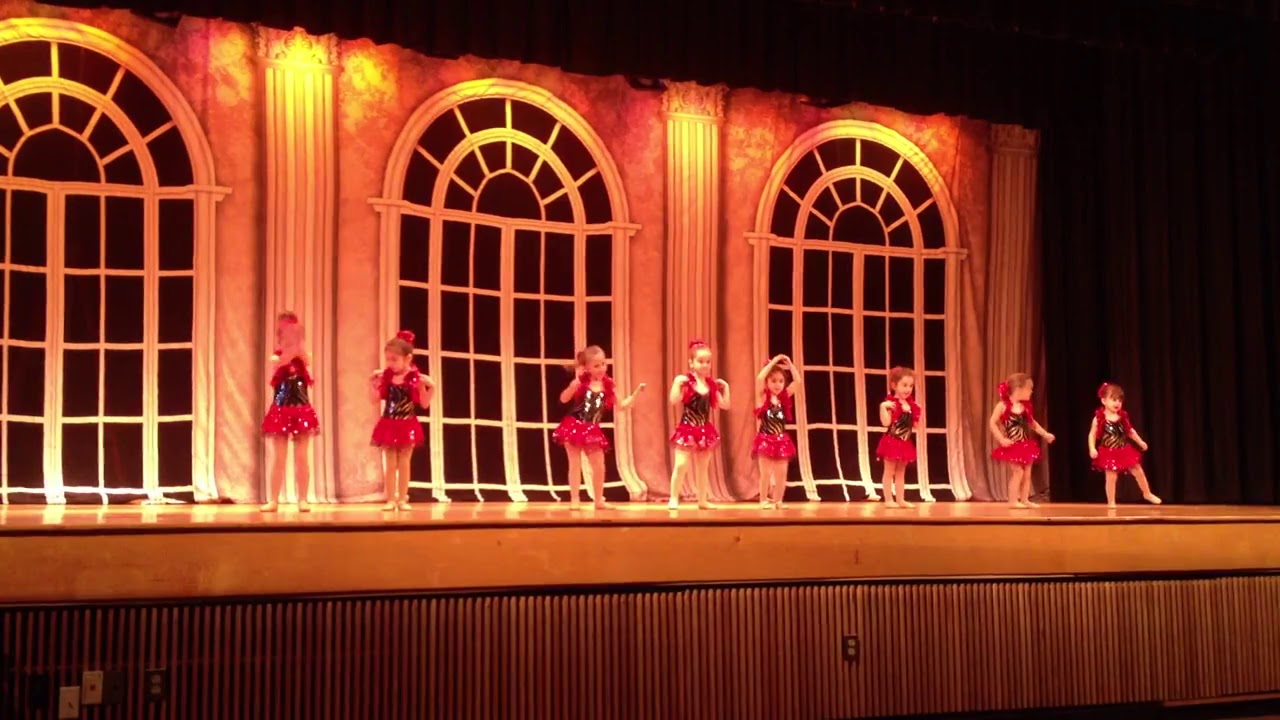In this image, eight young girls, likely around five to seven years old, are performing a dance on a wooden stage. They are dressed in coordinated costumes featuring sparkly black tank tops, short red flared skirts, and ballerina shoes. Their hair is adorned with cute red scrunchies or ribbons. The stage backdrop is designed to resemble a grand ballroom, with large arched windows and elegant columns, creating an atmosphere of sophistication. The girls are striking various poses, with some raising their arms and others shifting their feet in graceful dance moves. Electrical outlets are visible on the stage floor, adding to the authenticity of the setting. Overall, the scene captures a charming moment of a children’s ballet or theatrical performance, full of energy and elegance.